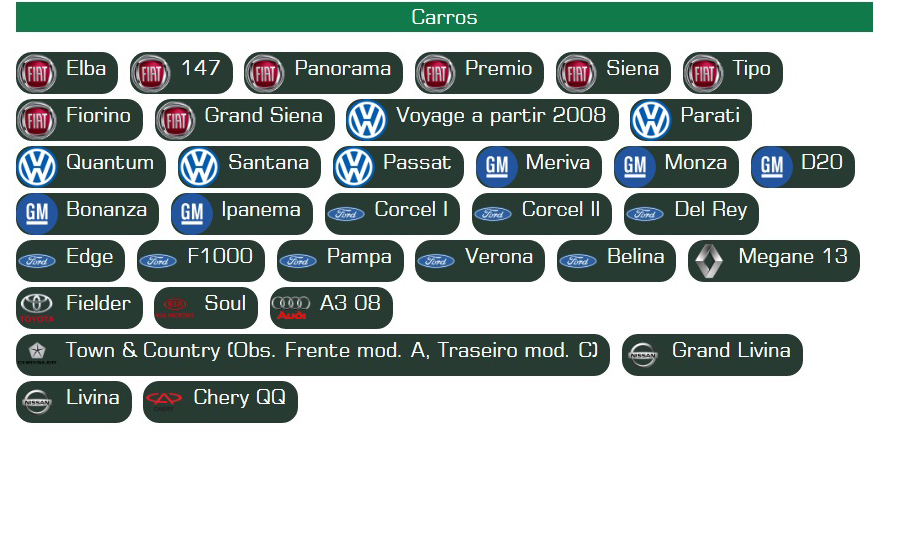This image features a structured chart of car names titled “Karros” in bold white letters on a dark green stripe running horizontally across the top. The background is predominantly white, interspersed with very dark green, rounded rectangular blocks containing car details. Each block lists a car make, followed by specific models or names. Starting from the top left, the first section showcases various Fiat models including the Elba, 147, Panorama, Premio, Siena, Tipo, Fiorino, and Gran Siena. The next section is dedicated to Volkswagen and includes models such as Voyage Apartir 2008, Parati, Quantum, Santana, and Passat. Following this, the General Motors section can be identified by a blue circle with a white GM logo and includes models such as Riva, Monza, Bonanza, and Ipanema. The Ford section lists models like Corsair 1, Corsair 2, Delray, Edge, F-1000, Tampa, Verona, and Berlina, marked by the iconic blue oval logo. Renault is represented by a silver diamond emblem, listing the Megane 13, while Toyota, denoted by its red logo, includes the Fielder. Additional make and models mentioned include Kia Soul, Audi A308, Chrysler Town and Country, Nissan Grand Livina, and Livina, and Jeep, culminating with Cherry QQ. The image appears printed digitally and features both emblematic car logos and specific vehicle names, creating a clear, organized visual reference for various automobile makes and their models.